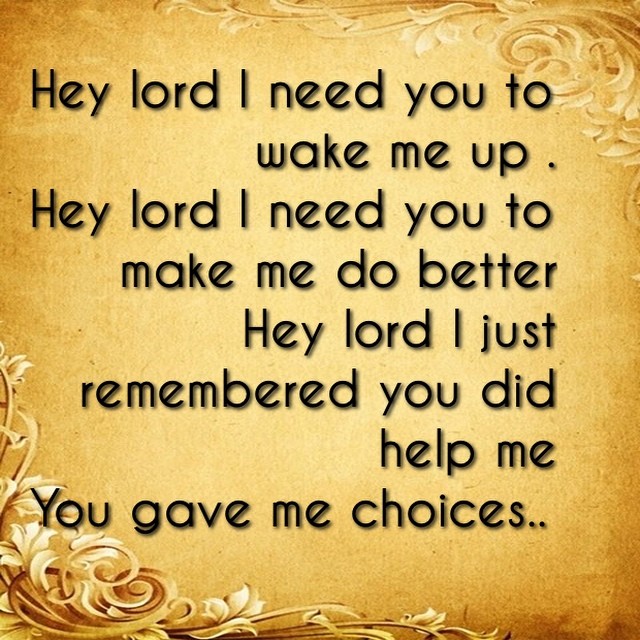This square image showcases an artwork with a quote overlaid on a bright gold and somewhat grainy background. The coloration transitions to a more brownish hue in the top left and bottom right corners. Adorning the top right corner is a faint gold design featuring swirls, petals, and flowers with hints of white and yellow, extending towards the top left. The bottom left corner displays a vivid, darker pattern with gold vines, swirls, and leaves, also accented with white and yellow. Black text with faint shadows spans the center of the image, presenting a prayer-like quote: "Hey, Lord, I need you to wake me up. Hey, Lord, I need you to make me do better. Hey, Lord, I just remembered you did help me. You gave me my choices..." The overall simple yet elegant composition, with its floral designs and golden backdrop, creates a visually appealing prayer reminder often shared on social media.